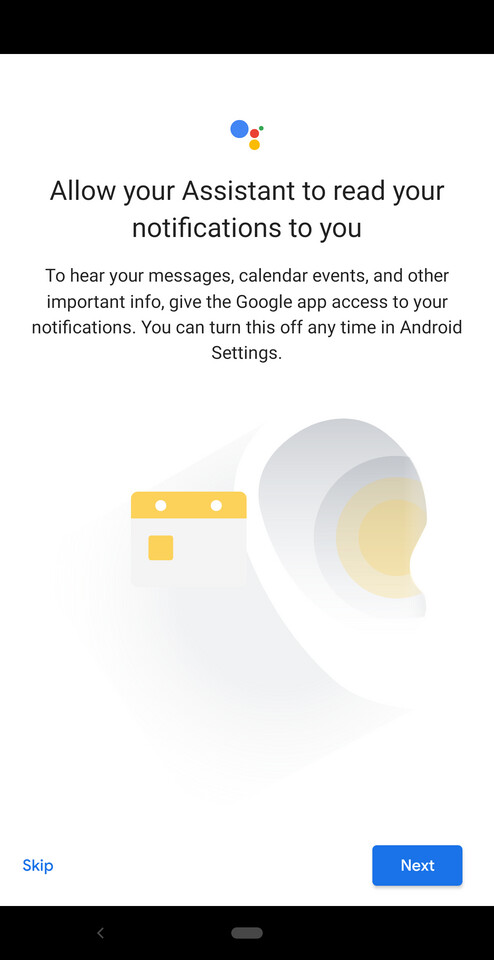A detailed descriptive caption for the image could be as follows:

"This image is a screenshot taken from an Android mobile device. It displays an informational pop-up from Google Assistant, prompting the user to allow the Assistant to read notifications, including messages, calendar events, and other important information. The pop-up is titled 'Allow your Assistant to read your notifications,' with 'Assistant' clearly capitalized, indicating Google Assistant. The message explains that the Google app requires access to notifications to carry out this function and assures users they can disable this feature any time in the Android settings. The visual aspect of the pop-up includes a minimalist icon: an ear, depicted with subtle gray shading on a white background. Next to the ear is a yellow calendar icon, with a yellow gradient circle emanating from the ear, symbolizing the audio reading of calendar events. At the bottom of the pop-up, there are two buttons: 'Skip' on the left and a blue-outlined 'Next' button on the right. This interface element emphasizes user choice, allowing them to proceed or dismiss the feature as they wish."